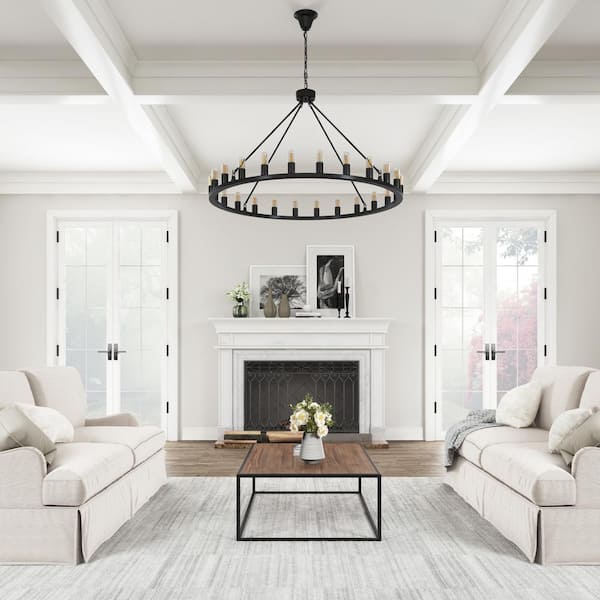The image portrays an elegantly designed living room adorned with a mix of neutral tones and subtle accents. Dominating the space, two cream-colored sofas, likely made of cotton, face each other on a light gray sectional rug featuring some white streaks. Centered between them is a square wooden coffee table with sleek black legs. Above, a black chandelier with multiple candle-like lights hangs from a chain, adding a touch of sophistication.

The room's walls and ceiling are painted in a crisp white, complemented by the gridlock of support panels that hang slightly below the main ceiling. On one side of the room, a white mantle fireplace is decorated with two black and white pictures and flanked by a pair of vases with flowers. This side also features double patio doors with white trimming, providing a glimpse of greenery and some pinkish hues from the outside.

The color palette consists predominantly of white, black, gray, and brown, with hints of yellow and green contributing to the cozy yet chic atmosphere. The room’s thoughtful arrangement and elegant decor suggest it could be featured in a high-end home decor magazine.